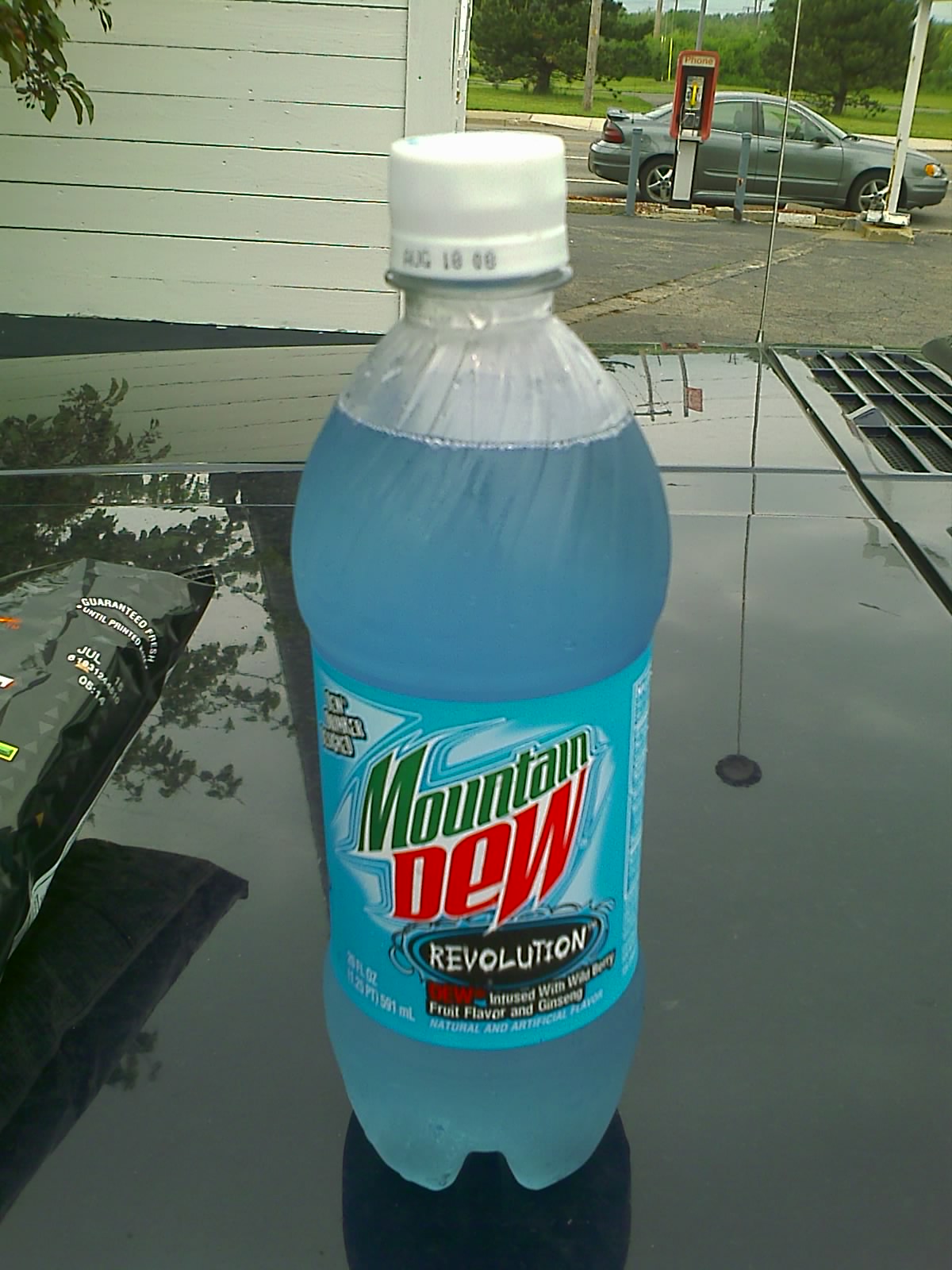In this close-up photograph, a clear plastic bottle of Mountain Dew Revolution, filled with a light blue liquid and capped with a white plastic top, is prominently featured. The bottle, beaded with condensation, suggests it's exceptionally cold. It rests on the shiny, black hood of a car, gleaming as if freshly waxed. To the right of the bottle, a car antenna stands out, while to the left, a black plastic bag lies on the hood. The backdrop reveals an asphalt parking lot where a gray sedan is parked beside an air tire pressure pump, adding context to the scene. This juxtaposition of the chilled soda bottle on the polished car hood against the everyday setting of a parking lot creates a striking visual contrast.